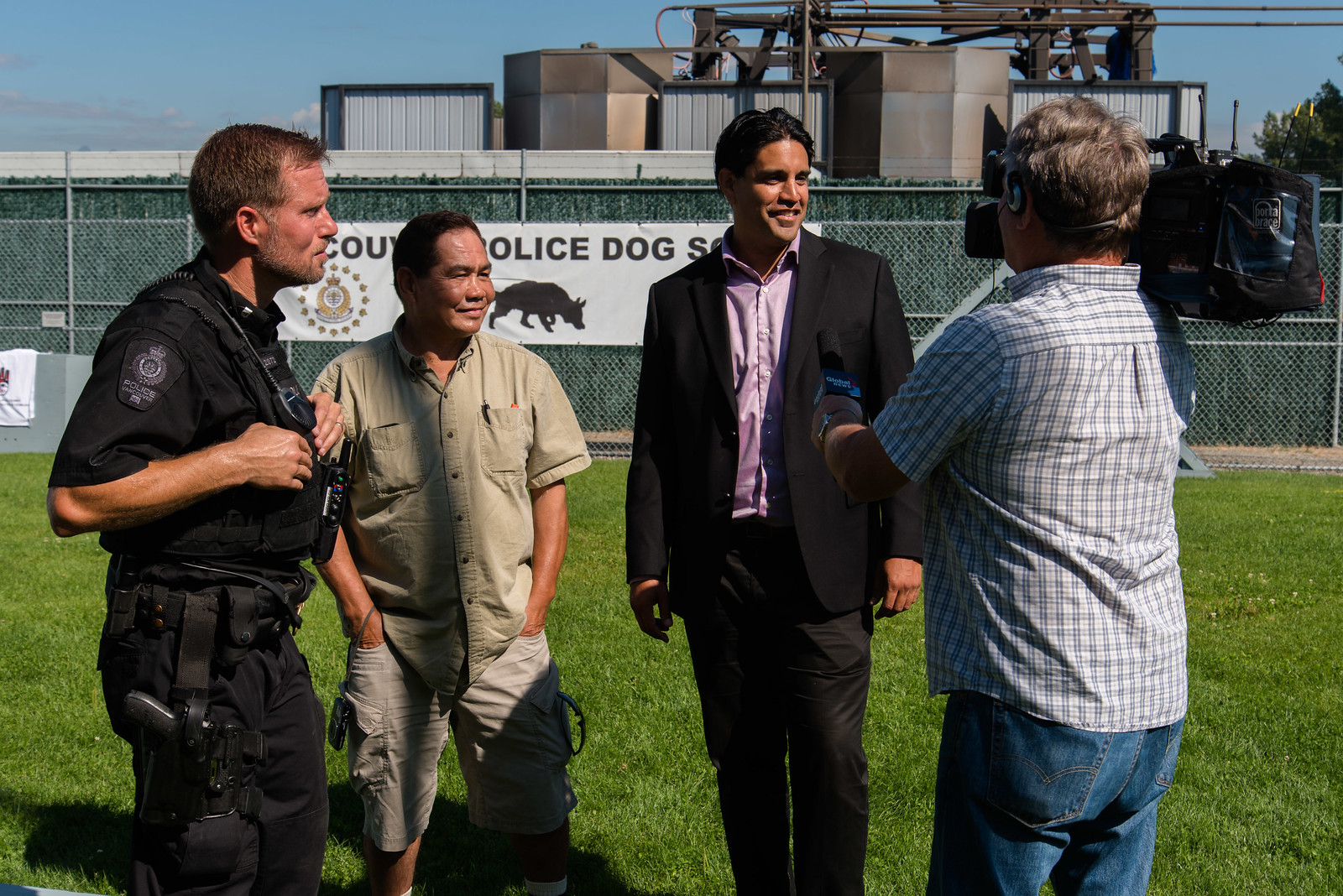In the photograph, a news team is conducting an interview at a dog training facility. The scene, bathed in daylight, is set in a grassy field enclosed by a wire netted barricade. Directly visible is a white banner with an image of a dog and the logo for "Police Dog School," along with some text likely indicating the facility's name. In the background are large industrial buildings, distinguished by their cylindrical and cubical structures.

Prominently featured in the photo are four men. On the far left stands a middle-aged police officer dressed in a black uniform adorned with various gear, including a police badge, belts, a walkie-talkie, and likely a firearm holstered at his hip. 

Next to him is an older, Asian man wearing a beige button-down shirt and khaki shorts. He has a small digital camera hanging from his wrist and sunglasses tucked into his shirt pocket. Both his hands are casually placed in his pockets.

In the center, engaging with the news team, is a man in a black suit, complemented by a light pink button-down shirt. He is smiling as he speaks, his expression professional and approachable. 

On the far right is the cameraman, easily identified by the large camera on his right shoulder and the microphone in his left hand. He wears a checkered light gray shirt and blue jeans, along with a wristwatch and headphones. The microphone bears the "Global News" logo, highlighting the professional nature of the interview. The cameraman's hair is a mix of brown and white, suggesting some age.

The overall impression is one of a well-coordinated interview taking place in a setting dedicated to police dog training, amidst the tranquility of a sunny day.